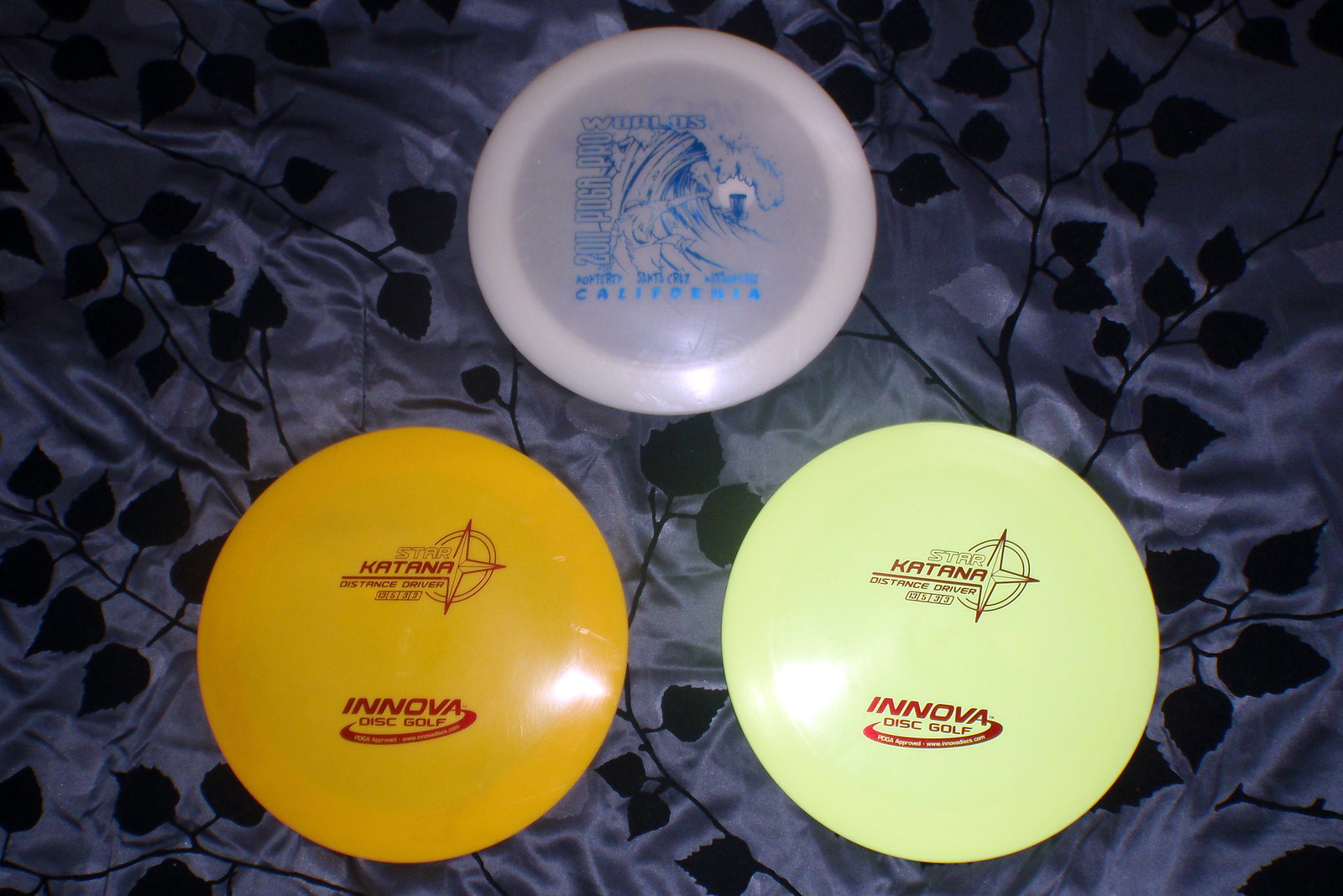The photograph showcases three Frisbee discs arranged in a pyramid formation on a dark blue, satiny comforter with an embroidered design of leaves. The top disc is transparent with a pink undertone and features blue text that reads "2011 Poga Pro" along with additional illegible words and "California." It has a wave-like logo. The bottom discs are both labeled as Star Katana Distance Drivers from Innova Disc Golf. The disc on the bottom left is mustard yellow, while the one on the bottom right is a light neon green. Both have similar designs with the word "Katana," a star logo, and the Innova branding.